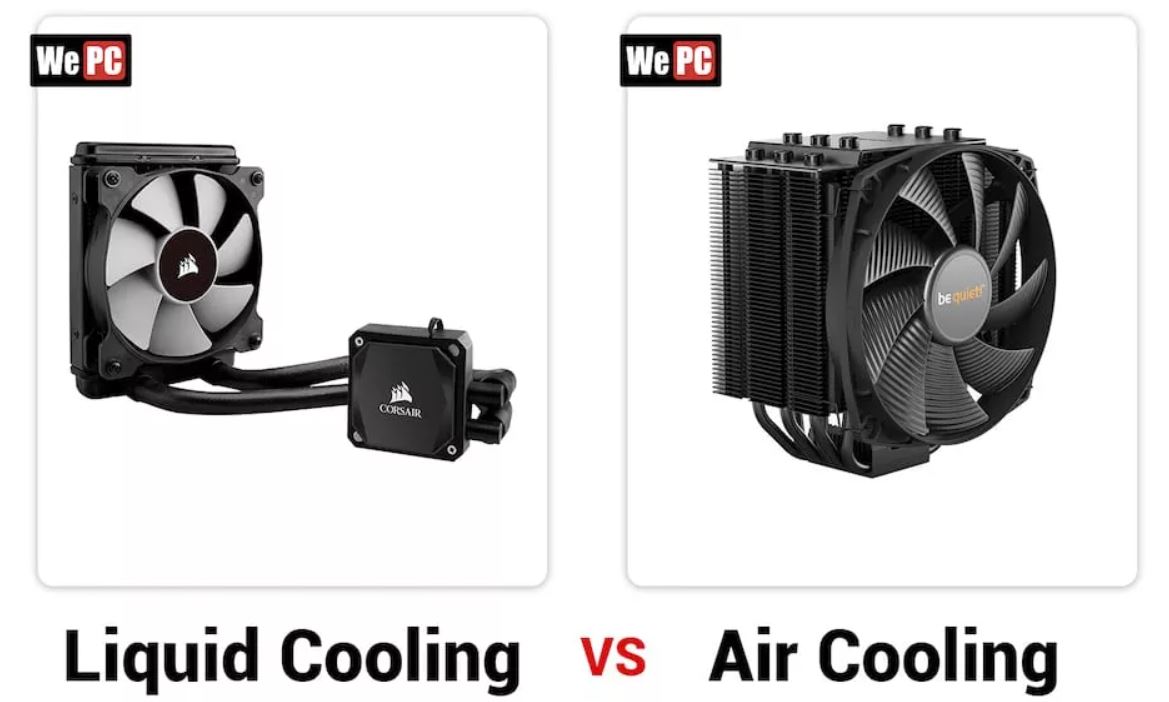The image is a detailed advertisement for WePC, showcasing a comparative analysis of two computer cooling solutions: liquid cooling and air cooling. The top of the image features the WePC logo prominently. The image on the left demonstrates the liquid cooling system, which consists of a smaller, more streamlined unit that includes a fan connected by two tubes to a compact black box branded with the Corsair logo. The caption beneath this unit reads "liquid cooling." On the right, the air cooling system is depicted as a larger and more complex mechanism, featuring a substantial black fan branded by Be Quiet. This unit is bulkier and has multiple tubes attached to the back. The image background is plain white, ensuring the focus remains on the products. At the bottom of the image, the text "Liquid Cooling versus Air Cooling" clearly indicates the intent to compare these two cooling methods, highlighting their physical and functional differences.